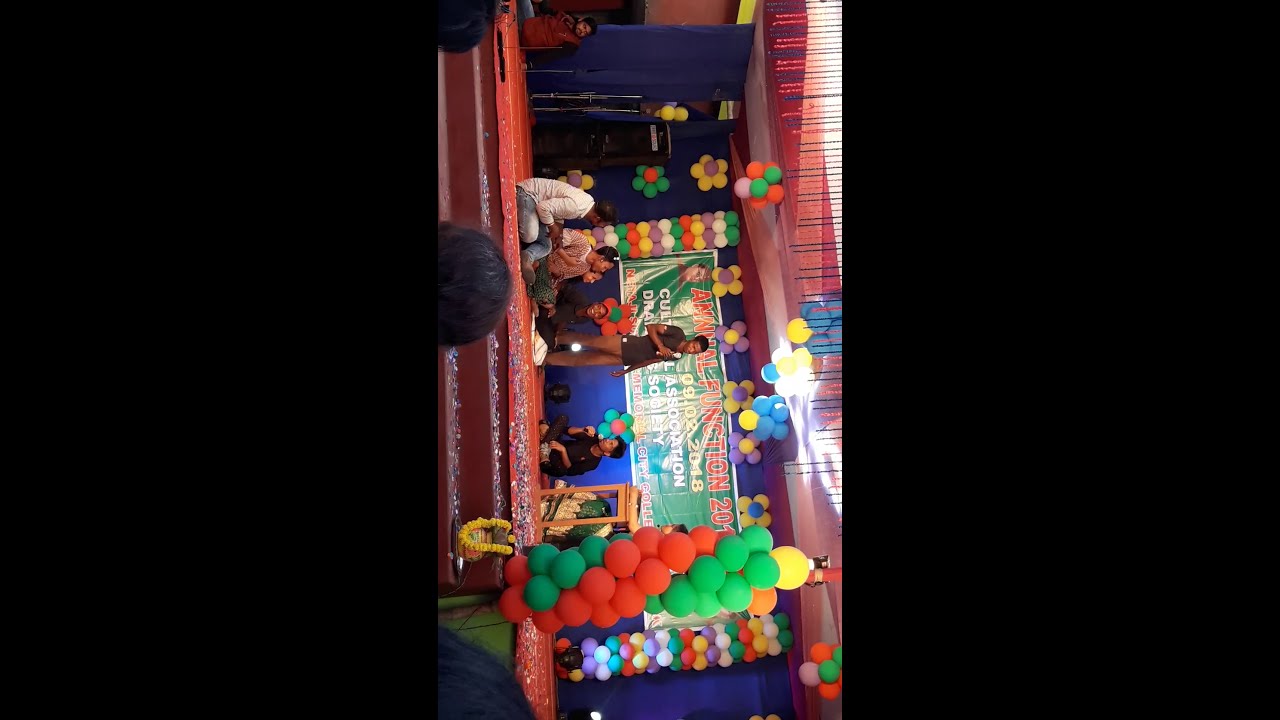This is a photograph of a vividly decorated stage, set for a children's show. The stage is predominantly red with a shimmery overlay. On it, five young boys are seated, some holding microphones, while a young gentleman stands in the middle dressed in a black short-sleeved shirt and black shorts. Clusters of multi-colored balloons – including green, orange, pink, yellow, purple, and blue – adorn the stage, with some hanging from the ceiling and others gathered in netting on the sides. A large green banner with red and white letters hangs in the background, displaying "Annual Function 2018" and the date "09-02-2018," representing the Cultural Association. The stage also includes three steps leading up to it. The image appears to have been captured sideways with a smartphone, which gives the stage a vertical orientation.